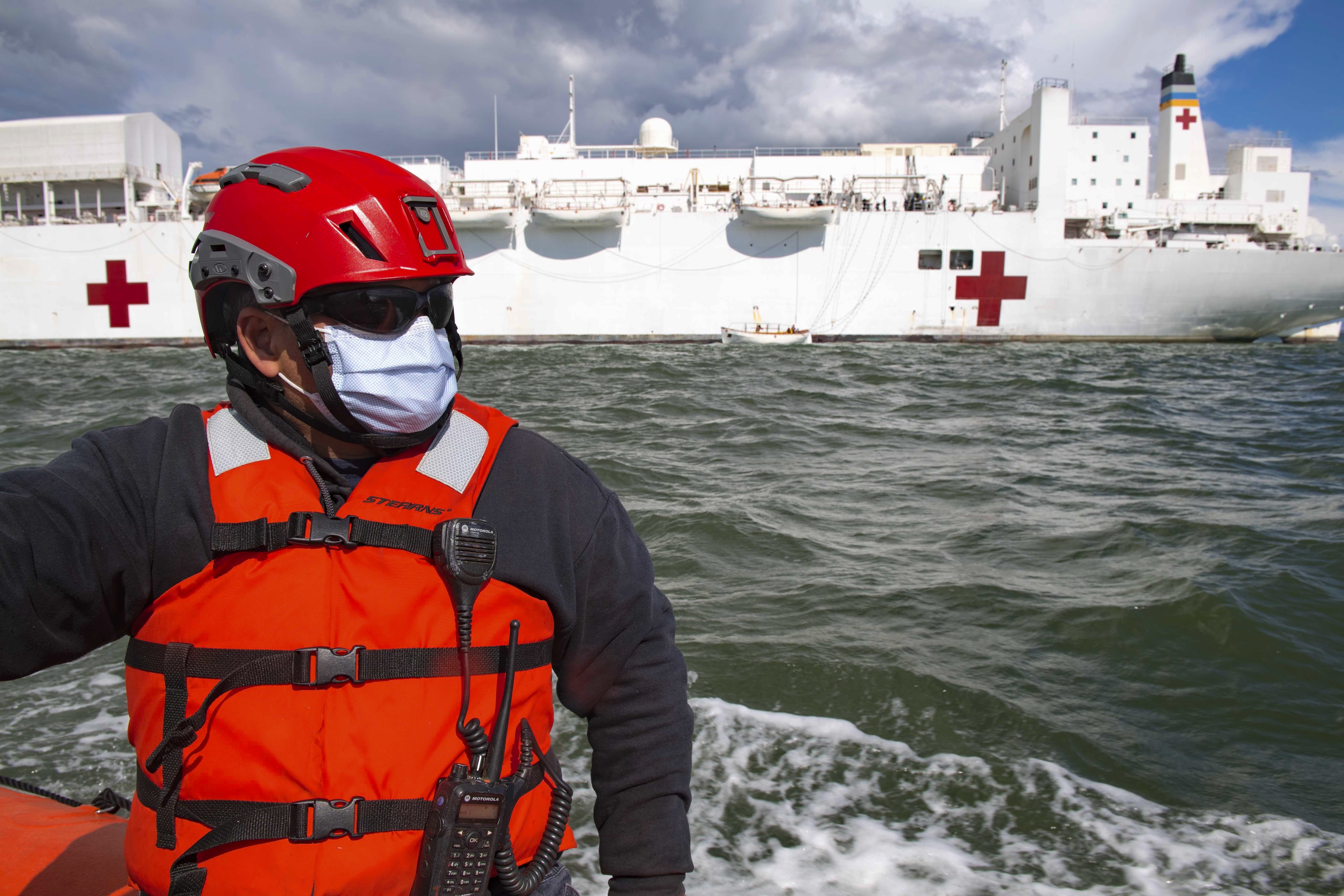The image depicts a scene set in the ocean during the day, featuring a man in the foreground sitting on a bright orange lifeboat. The man is equipped for safety with a red helmet, a face mask resembling those used during the COVID-19 pandemic, black sunglasses, and a bright red life vest with a walkie-talkie clipped to it. He is also wearing a long black sweater. The background prominently displays a massive, white hospital ship adorned with two large red crosses. The ship dominates the background, with the sky showing some sun and clouds, and the ocean waters appearing relatively calm. In the distance, a considerably smaller white lifeboat with people onboard can be seen, suggesting a potential rescue mission or transit to the larger ship.